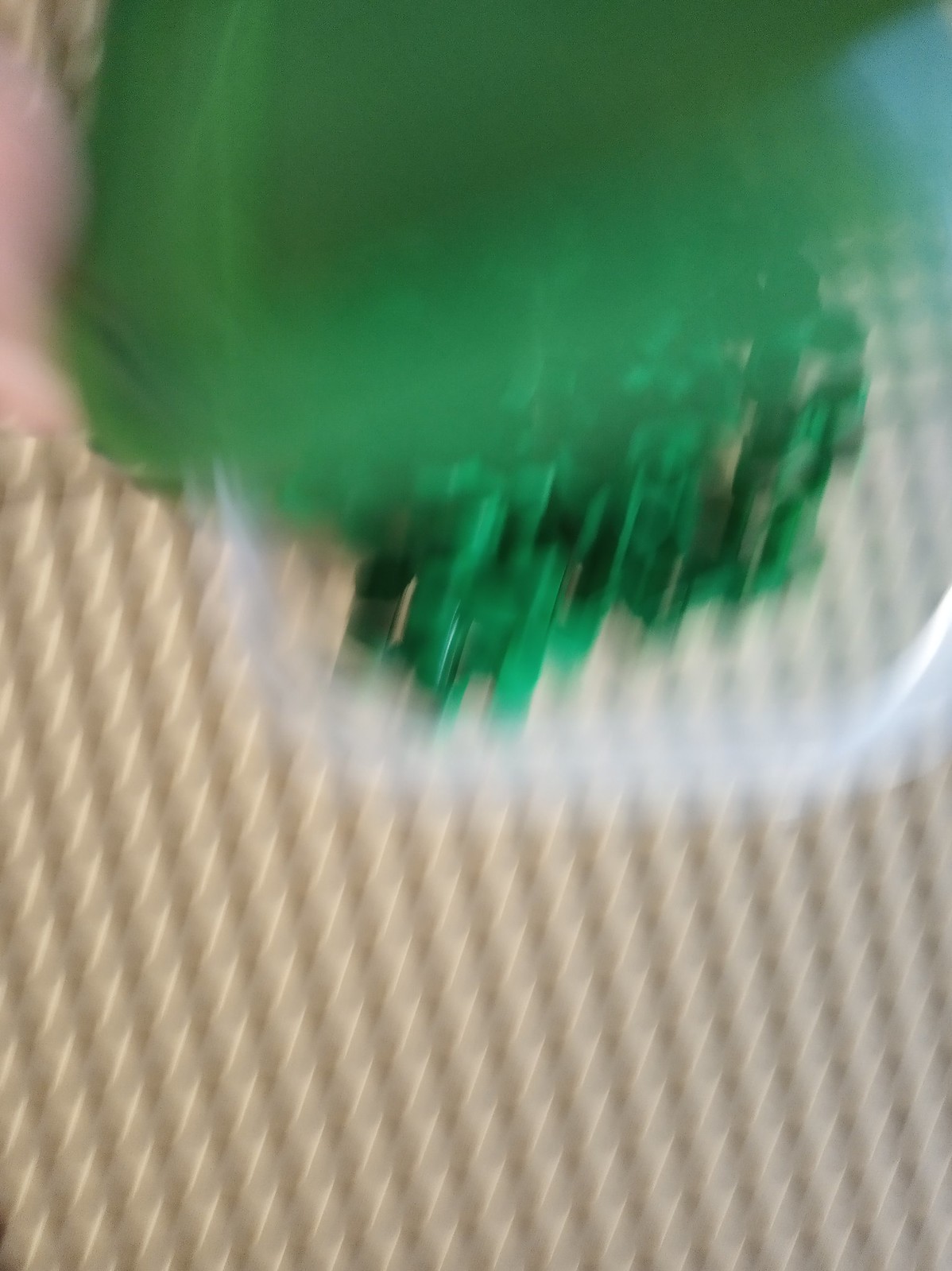The image is an up-close, very blurry color photograph with a rectangular orientation, where the larger side is vertical. The photograph is essentially divided into two distinct sections. 

The bottom portion of the image showcases a zoomed-in view of pink fabric, detailed with individual small circles arranged in rows, separated by darker pink, slightly diagonal lines slanting to the left. In this section, there are coils of beige or tan fabric interwoven with lighter threads, appearing as vertical ribbons tilted slightly to the left. A white thread meanders through these shapes, giving it a textured appearance.

Transitioning to the upper half of the image, there is a solid green mass, likely dark green in color, with a description that suggests it might be a fabric or package. This area features a slight diagonal element coming from the top left, described as a thin outline or bar that curves over and extends off the right side of the frame. At the top right corner, there's a small blue spot, adding a bit of contrasting color to the otherwise green and pink hues. The green fabric appears dense, with its bottom half showing blurrily rendered tentacle-like extensions or shapes.

Overall, the photograph captures a detailed yet indistinct assortment of colors and textures, emphasizing pink and green fabrics interspersed with tan and white threads, all rendered in a highly blurred and abstract manner.